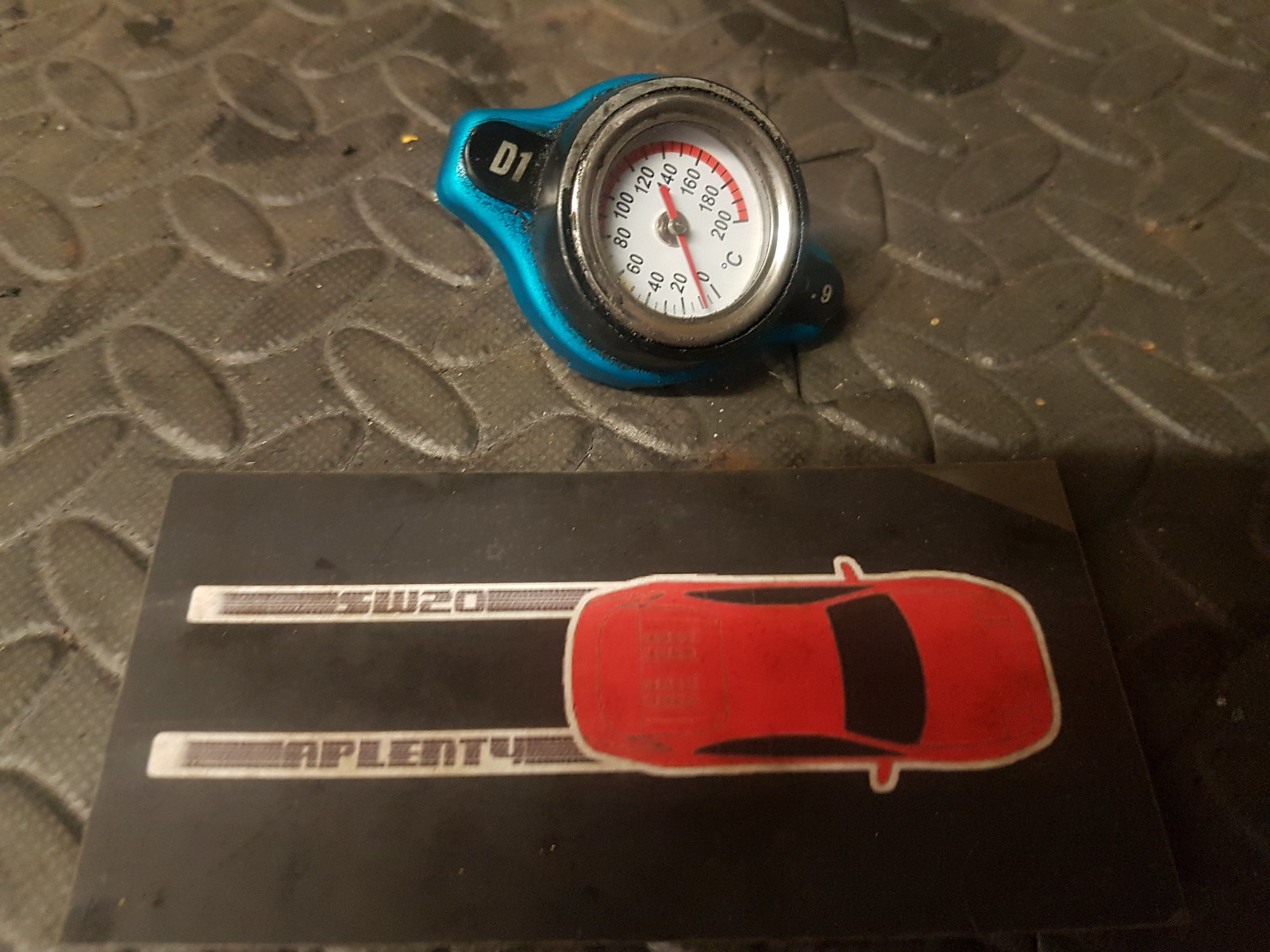This photograph, captured in landscape mode, offers an intimate, close-up view of the cluttered top of a workbench, likely situated in an automotive garage. The image features two distinct objects set against the textured background of the workbench.

The first object is a tire pressure gauge, characterized by its predominantly round shape and blue exterior. The gauge's display screen prominently features the alphanumeric marking "D1" above it. Interestingly, the display shows a temperature readout in Celsius, ranging from 0 to 200 degrees, though the specific application of this measurement remains unclear. Additionally, the number "0.9" is displayed outside of the main readout, further adding to the intrigue of its function.

In the foreground, there is a black box with a clipart-style image of a red car viewed from above. The car is depicted with a black windshield and side windows, seemingly in a skidding motion. The top skid mark in the illustration bears the label "SW20," while the bottom skid is inscribed with the word "aplety" (A-P-L-E-N-T-Y). This combination of elements enhances the automotive theme of the workbench setting, suggesting a possible connection to vehicle maintenance or diagnostics.